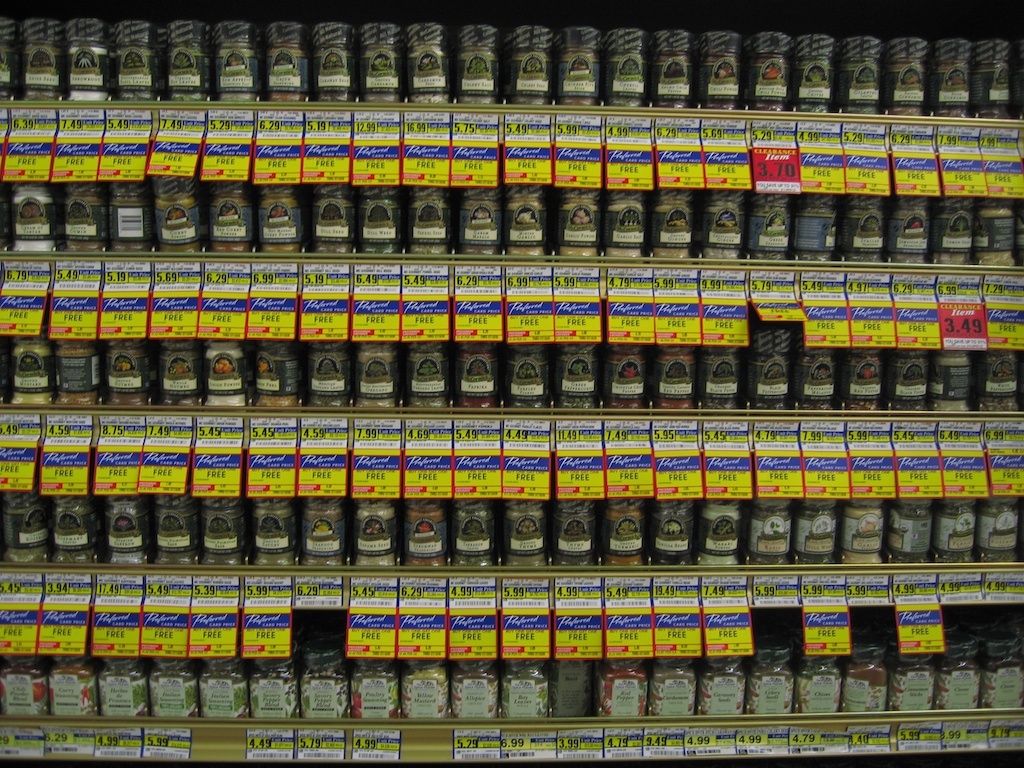The image depicts a store shelf dedicated to a variety of spices and seasonings. The shelf is tiered, consisting of five levels stacked with different spice jars and containers. Prominently, the top level showcases several seasonings, each accompanied by its price indicated with yellow tags, suggesting these items are currently on sale. Notably, in the upper left-hand corner, the prices range from $5.29 to $7.49. Specifically, one seasoning is priced at $6.39, another at $7.49, followed by one at $5.49, then another at $7.49, and finally, one at $5.29. The vibrant yellow tags hint at "buy one get one free" offers, making these spices not only essential for culinary use but also a good deal for shoppers.